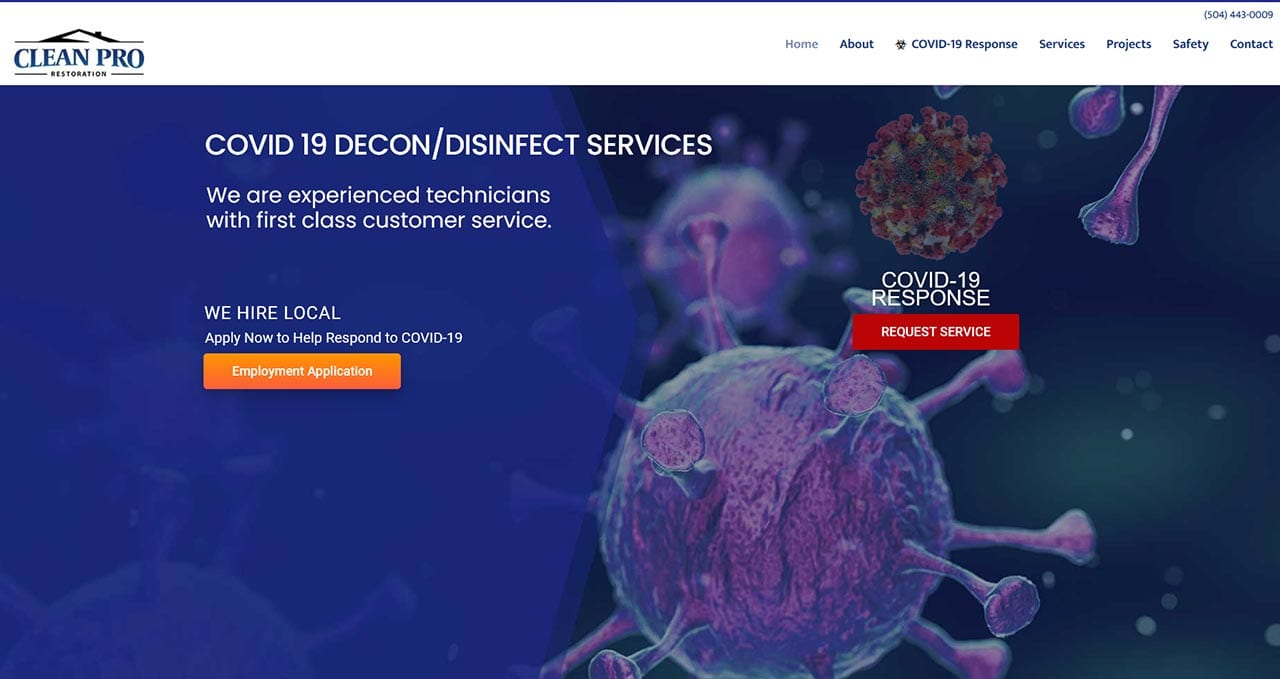Screenshot of Clean Pro Restoration's Webpage

The featured image on the webpage is a vivid illustration of the COVID-19 virus, depicted in striking blue with purple highlights and distinctive spiky protrusions encircling its round core. The virus stands out prominently against a dark gray, almost black, background, creating a stark and impactful visual.

Centered on this background is the phrase "COVID-19 Response," accompanied by a bold red button labeled "Request Service." To the left of the virus image, white text announces "COVID-19 Decon/Disinfect Services" followed by a brief description: "We are experienced technicians with first-class customer service. We hire local."

Below this message, an orange button with white text invites users to "Apply now to help respond to COVID-19," and an adjacent prompt to "Employment Application" for those interested in joining the team.

This webpage is a clear and compelling call to action for both service requests and employment opportunities, encapsulated within a professional and visually engaging design.